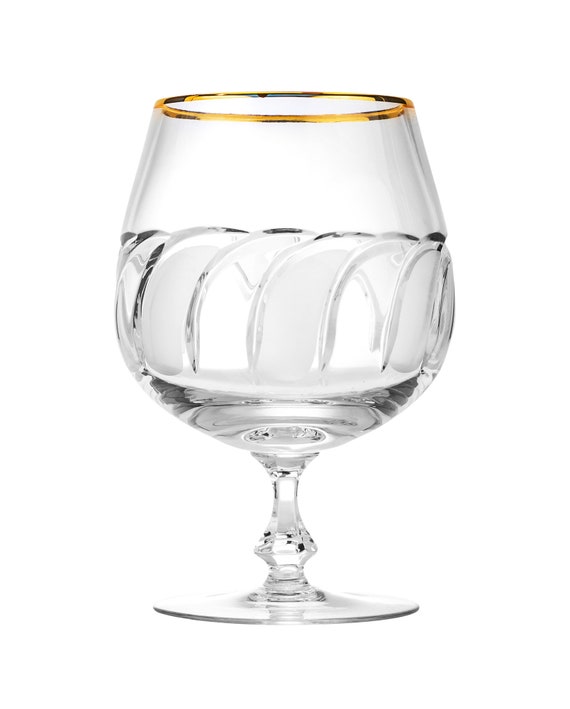This photograph captures an elegant glass set against a solid white background, which dominates the majority of the space. The glass itself, designed for cognac, features an elegantly curved silhouette. It widens at the bottom and narrows as it nears the top, creating a refined and classic shape. The stem of the glass is broader at the base and tapers gracefully. The base and the rim, which is adorned with a ring of gold, are roughly the same size, contributing to a balanced aesthetic. This rim, where one would place their lips, adds a touch of luxury. Midway up the glass, there are curving lines that form a decorative pattern, adding a subtle, yet sophisticated ornamentation. Despite its ornamental details, the design retains a sense of simplicity, avoiding stark modernist minimalism while maintaining elegant sophistication.